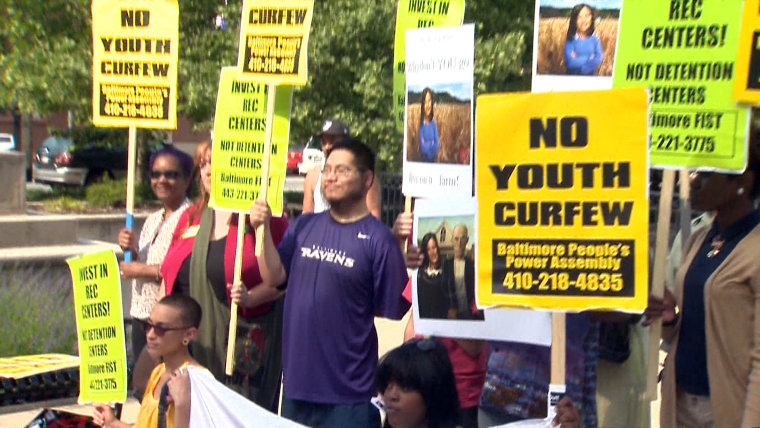This slightly blurry, full-color photo captures a vibrant and diverse protest in Baltimore, Maryland. The crowd is united against the proposed youth curfew, holding up various signs, the most prominent of which declares, "No Youth Curfew." This sign is accompanied by another that reads, "Baltimore People's Power Assembly" with the contact number 410-218-4835. Another notable sign states, "Rec Centers, Not Detention Centers!" emphasizing the community's demand for recreational spaces over internment-like facilities. Among the protesters, a mix of races and ages is evident, with some individuals smiling and others holding serious expressions. A man in a dark blue Baltimore Ravens t-shirt stands out, reinforcing the local context. Additionally, there are posters featuring an image of a young girl with folded arms, symbolizing the innocence and resilience of the youth at the heart of this issue. Some protesters are seated, holding a large yet partially obscured banner, further contributing to the sense of community and solidarity in this movement.